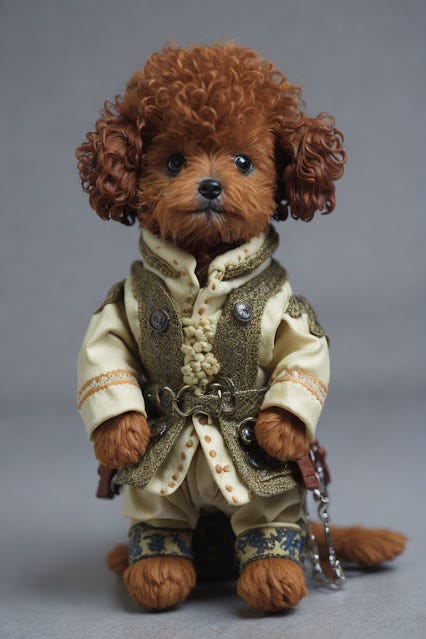This image portrays a detailed and elegantly dressed stuffed animal resembling a brown poodle with curly, afro-like fur concentrated on its head and ears and shorter fur on its snout. The toy stands upright on its hind legs, balanced like a human. It has dark eyes and a small black nose. The attire is a striking, old-fashioned ensemble, featuring a white, ornate high-collared shirt underneath a pale green vest secured by four large buttons. The shirt is complemented by a green trim on the collar and shoulders, and gold decorations on the wrists. The pants are adorned with vivid blue and gold patterns near the cuffs, adding to the intricate nature of the outfit. An elegant silver pocket chain drapes from the left hip, completing the ensemble and giving the stuffed poodle an air of vintage sophistication.